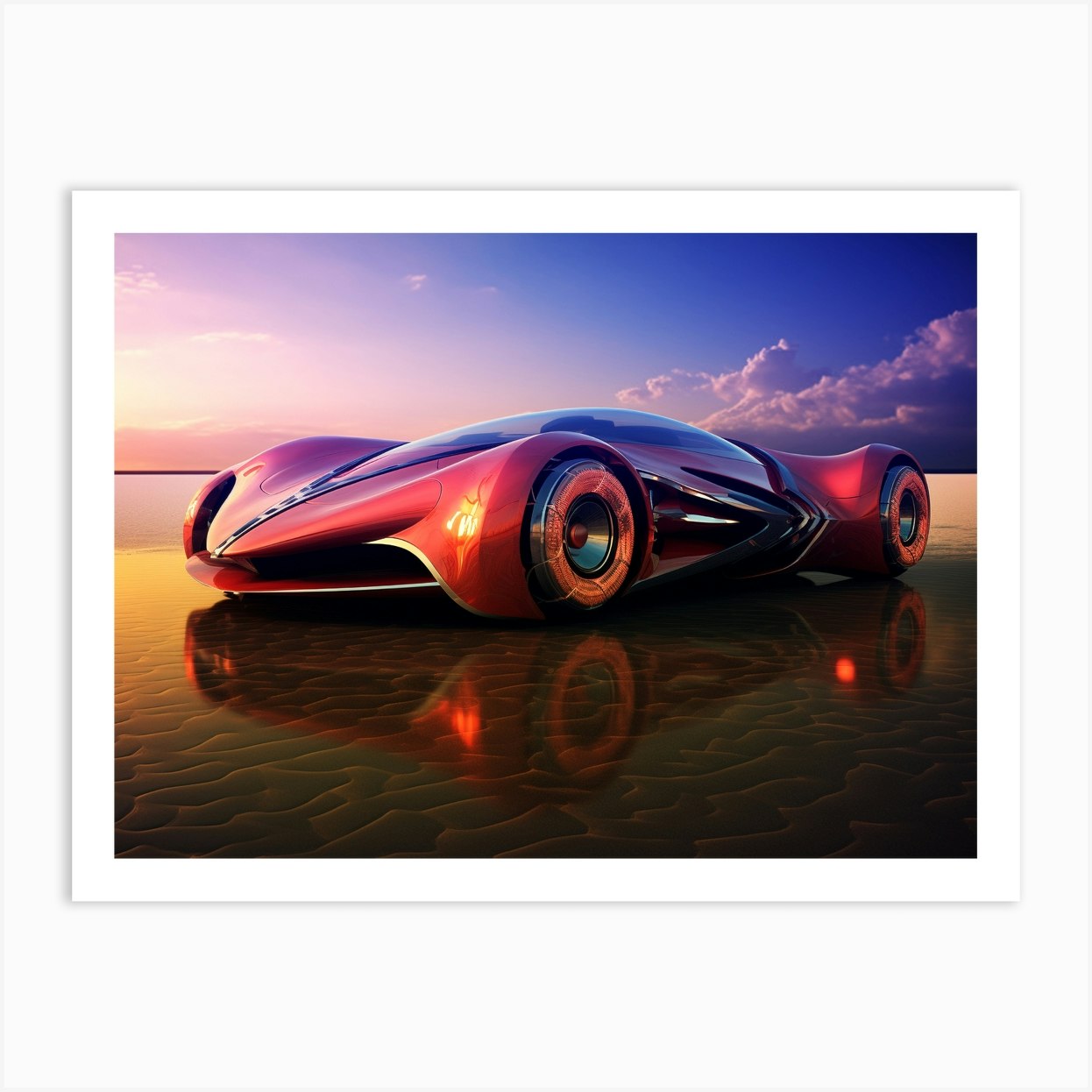The image is a detailed digital artwork of a futuristic, flat, and low sports car with smooth, fluid body contours. The car, which is predominantly a reflective bright red with some pink, purple, and orange highlights, is equipped with fancy chrome wheels that have red centers. Its design features a rounded sheet of glass at the top, resembling a bubble. The front of the car is narrow with a black grill resembling a mouth, while its doors are a sleek metallic dark gray. The wheels are a combination of black and orange, with shiny, red-accented hubs. The car appears to be sitting on a mirror-like, glassy surface that reflects its image, giving the impression of a reflective golden sand or shiny beach with grooves and patterns. The background includes a blue sky with fluffy white clouds, some grayish and pink-purple gradients, and a hint of sunlight streaming in from the left side, casting a warm yellow-green light. The entire scene is enclosed within a white frame against a white wall, emphasizing its polished and highly futuristic aesthetic.